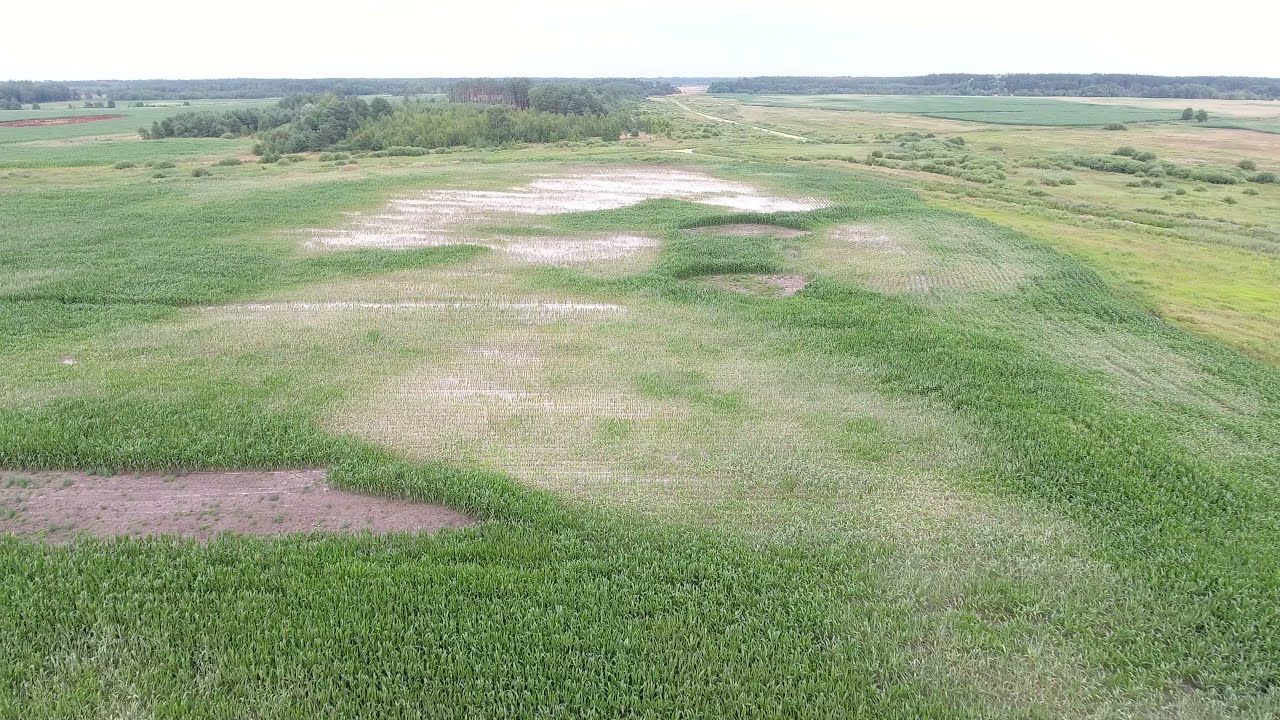The photograph is a horizontally aligned rectangular image of a field, taken from an aerial perspective that is not too high. The field is a blend of dark green, lighter green, and brown patches, depicting mixed vegetation and bare areas. The upper background is lined with dense rows of trees with green leaves, but no sky is visible. In the center-top third of the image, there is a bald, patchy spot with light brown gravel or whitish sand. Further blending into the field, from the middle to the bottom right, the vegetation thins out, showing more brown patches interspersed with green. A distinct strip of darker green runs across the bottom left towards the middle of the field. While there appears to be a dirt path or road in the upper center, there are no signs of people, vehicles, or buildings. The vegetation seems to include grass and possibly corn plants. The scene is an outdoor, daytime setting dominated by green, brown, beige, and whitish colors.